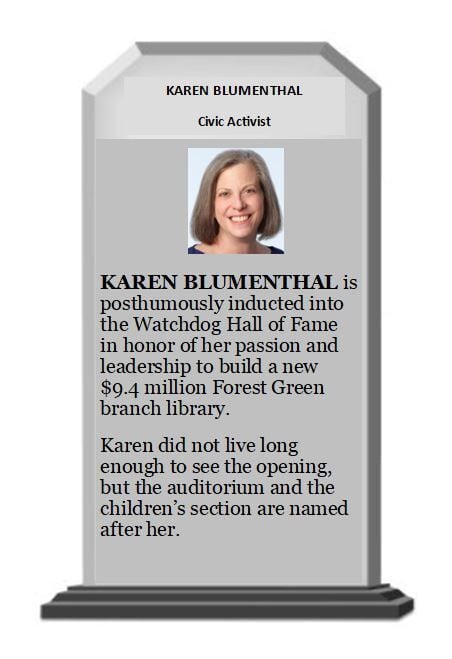The image depicts a cartoon-like memorial of Karen Blumenthal, a notable civic activist. It resembles a gray tombstone set against a white background. At the top of the tombstone, in black text, her name, "Karen Blumenthal," is inscribed, followed by the title "civic activist." Beneath this is a small photograph of Karen, a smiling woman of Caucasian European descent, in her mid to late 40s. The text below the photo reads: "Karen Blumenthal is posthumously inducted into the Watchdog Hall of Fame in honor of her passion and leadership to build a new $9.4 million Forest Green Branch Library. Karen did not live long enough to see the opening, but the auditorium and the children's section are named after her." The monument is digitally illustrated, and all the information is clearly presented in black lettering.